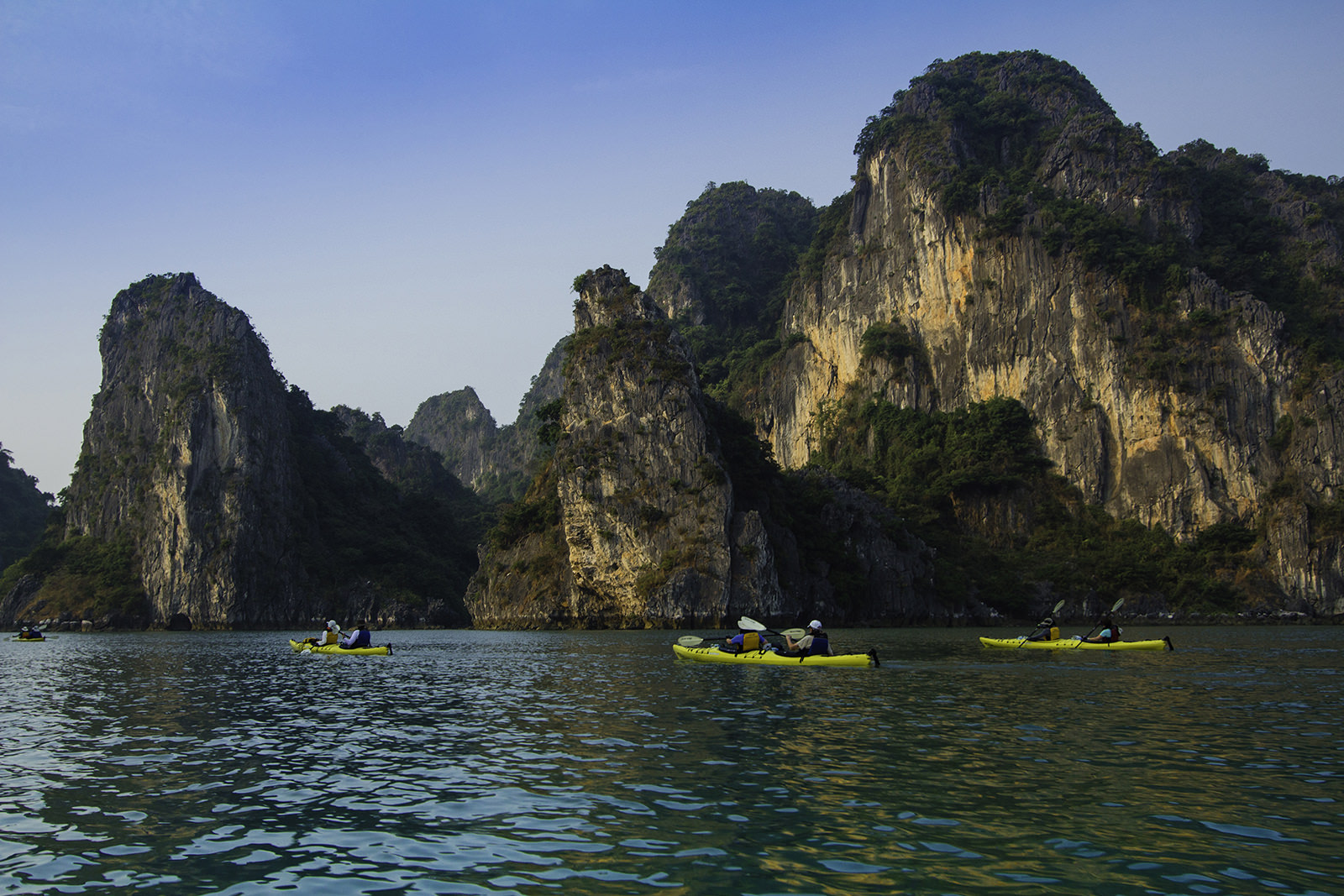This vivid and detailed landscape photo captures a serene scene of a calm lake surrounded by tall, rocky mountains. The mountains are predominantly brown-gray with some orangey highlights, and their steep cliffs are densely covered with green trees, grasses, and bushes. The still water in the foreground mirrors the hues of the mountainous terrain, creating a harmonious blend of colors. The clear, light blue sky above shows no clouds, adding to the peaceful ambiance. Closer to the middle ground of the photo, three groups of kayakers are navigating the water in bright yellow double kayaks. Each kayak has two people with black paddles featuring yellow blades, contributing to the vibrant and dynamic elements of the scene. The perspective suggests the photo might have been taken from another kayak, imparting a sense of immersion in this picturesque and tranquil environment.